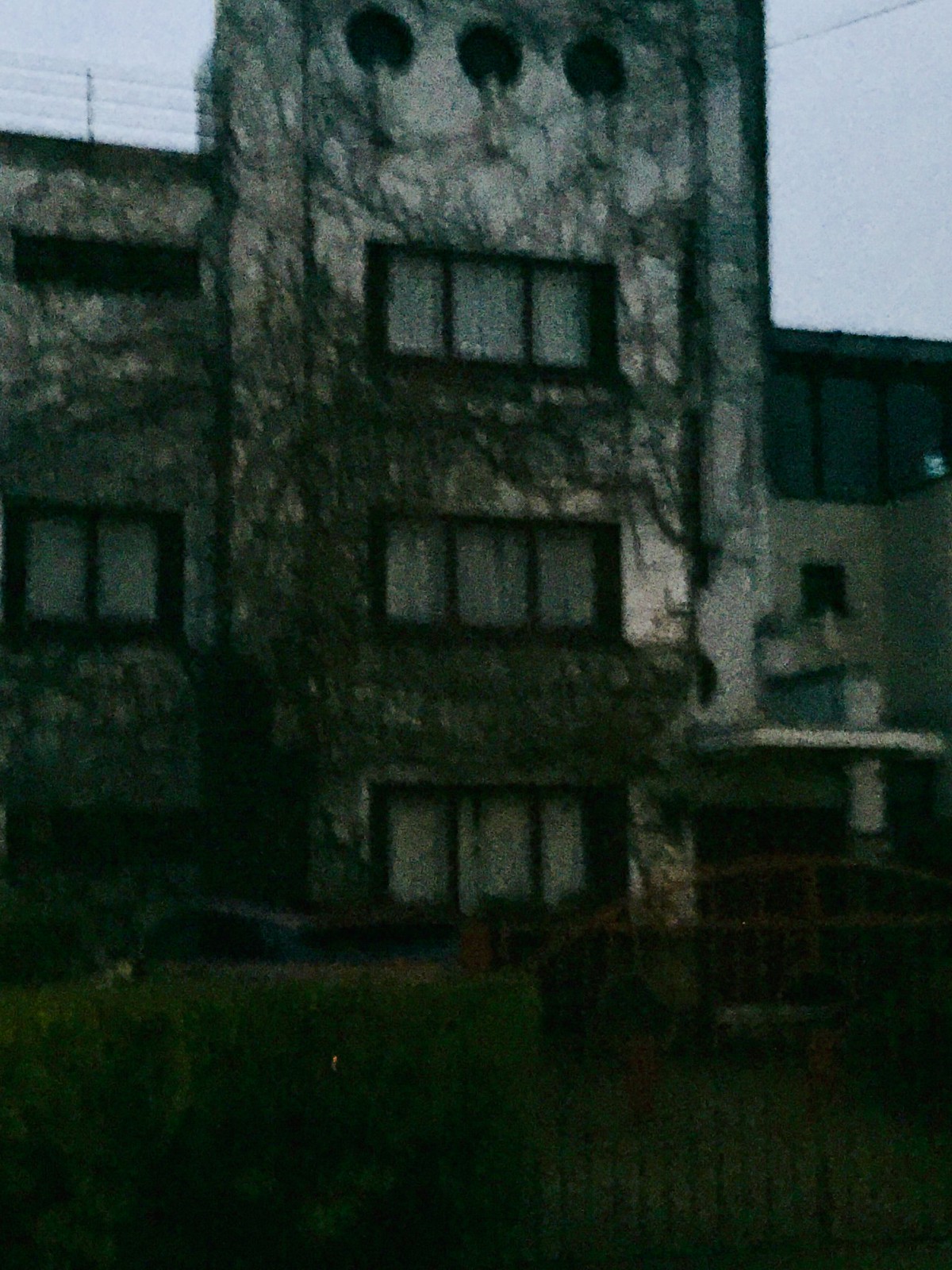This image showcases a desolate, three-story historic building, partially shrouded in bare, leafless vines. The structure features a prominent tower-like facade on the right side, encompassing three rows of windows, while adjacent sections of the building have a single row of windows each. A noticeable awning, possibly marking the entrance, is also visible. The building, rendered in a white, chalky hue, seems abandoned and weathered, surrounded by an aura of neglect. Above, the overcast, wintry sky hints at recent rain, adding to the somber atmosphere. The foreground is an expanse of unkempt grass, leading to a large, dark area at the base of the building, which appears to be the main entrance doors.